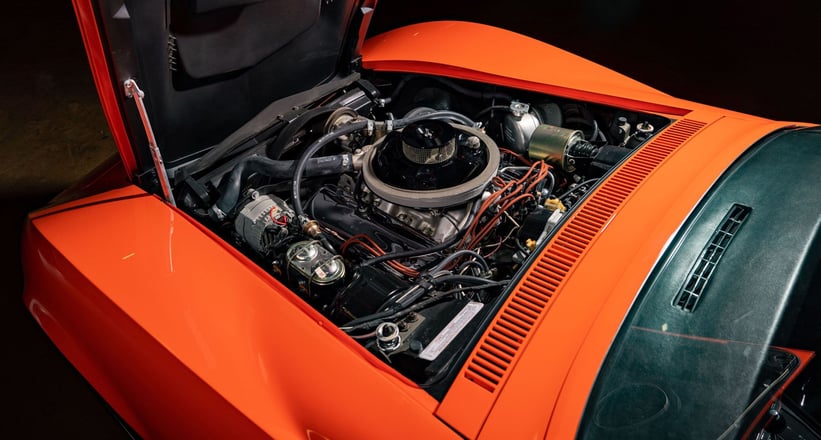This detailed photograph showcases the engine of a high-performance sports car, likely a Corvette or Camaro, with its bright orange paint job standing out prominently. The car’s hood is uniquely hinged at the front rather than the windshield, and it is open, exposing the engine. The image is captured from an overhead angle, looking down from the windshield area, providing a clear view of the engine compartment. The engine is a mix of silver metal fixtures, dark gray to black tubes and hoses, and orange wiring that matches the car’s exterior. Key components like a circular air filter, alternator, and distributor cap suggest it might be an older model. The photo appears to be taken indoors, possibly in a dark garage, given the black background that obscures the rest of the car and its surroundings. The image highlights the detailed, intricate design of the engine while giving a glimpse of the car’s partially visible dashboard through the windshield.